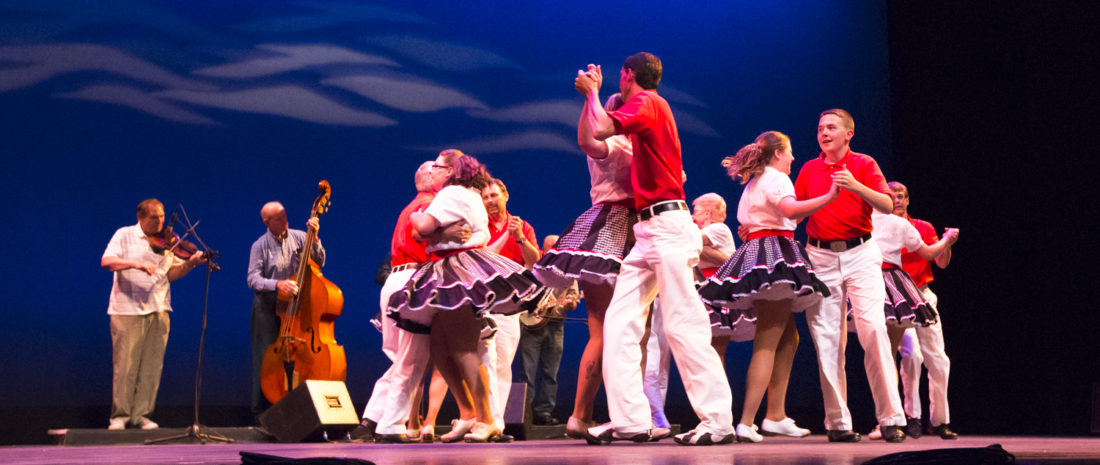The photograph captures a lively square dance performance on stage, set against a backdrop of what resembles a sapphire blue sky adorned with dolphin-like shapes or clouds. The male dancers are dressed in red tops paired with white pants, while the female dancers don vibrant purple and black petticoat skirts that flare dramatically when they spin, complemented by white tops and shoes. The dancers are closely paired, showcasing dynamic and synchronized movements. In the background, a small ensemble of musicians enhances the performance: one person on the right plays a large cello, another on the left handles a violin, and an additional figure is seen playing the guitar. The intricate details of the dancers' costumes and the festive ambience evoke the traditional charm of a square dance.